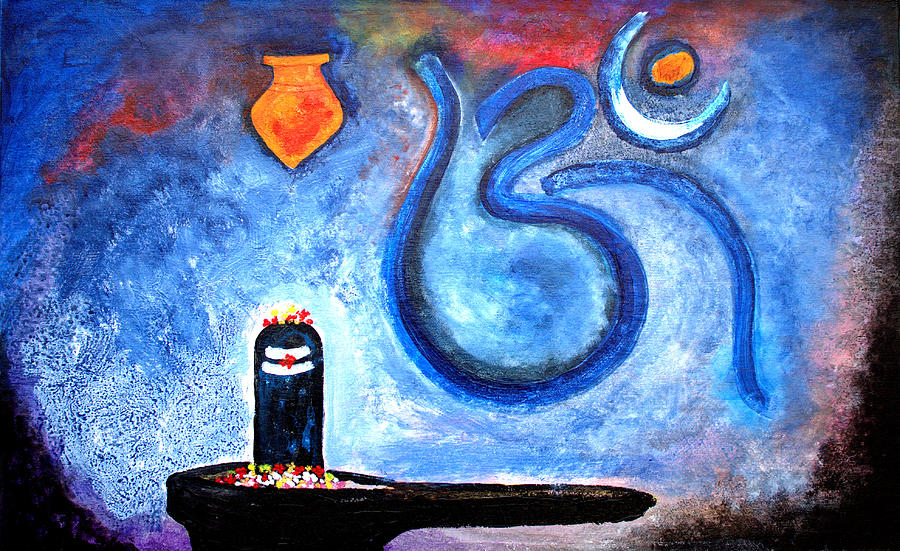The image is an abstract chalk drawing featuring a variety of seemingly unrelated objects against a dark and light brown background with shades of violet, deep blue, and orange. Central to the composition is an orange clay pot situated in the upper left-hand corner, resembling a terracotta planter or vase. Below, there appears to be a dark brown clay pan with a handle, positioned to the right, possibly representing a spoon or a similar kitchen utensil. This pan seems to contain white, orange objects—possibly flowers or pills. On the bottom left is a black totem figure rising from a colorful array of yellow, pink, white, and red flowers, topped with additional yellow and red blooms. Above these elements, a blue, circular squiggle, much like an incomplete ampersand, arcs towards a crescent moon. An overall dark border frames the bottom edges, enhancing the earthy tones and adding depth to the abstract scene.